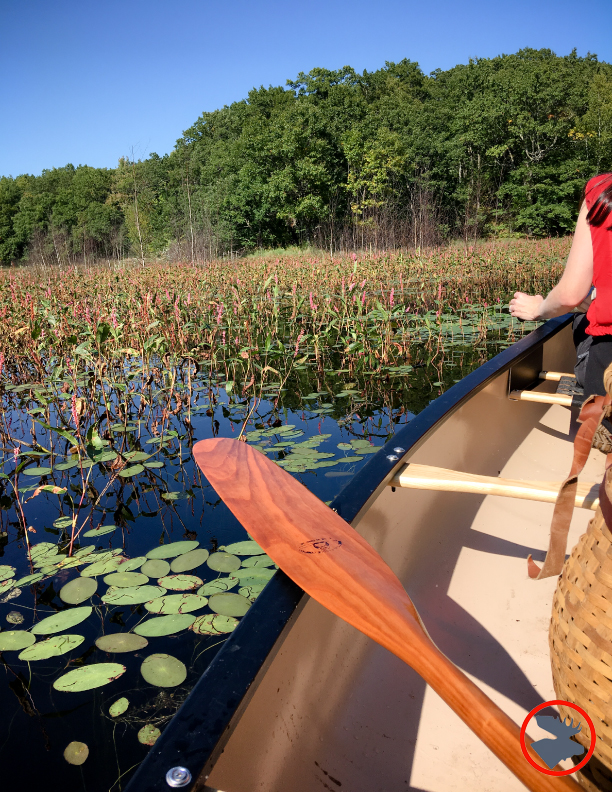In this picturesque image, a serene scene unfolds under a radiant blue sky dotted sparsely with fluffy white clouds. Towering trees frame the background, their lush, green foliage providing a serene canopy that hints at the outskirts of a dense, mystical forest. The landscape below is dominated by a vast, tranquil swamp, its glassy water surface festooned with clusters of vibrant green lily pads, offering a rich texture to the marshy expanse.

At the heart of this natural tableau is a boat gently drifting on the calm waters. The boat features a prominent black rim, contrasting with its light brown interior. Standing confidently at the bow is a person adorned in a sleeveless red shirt and dark pants, poised and seemingly in harmony with the peaceful surroundings. Light-colored seats span across the boat, offering glimpses of comfort and utility. A medium brown wooden paddle lies nearby, hinting at recent use or preparatory readiness.

Positioned to the side within the boat is a large woven basket, its rustic charm amplified by a substantial strap draped over its front. The basket hints at a purpose, perhaps for collecting specimens or carrying supplies, adding an element of intrigue and functionality to this tranquil outdoor snapshot.